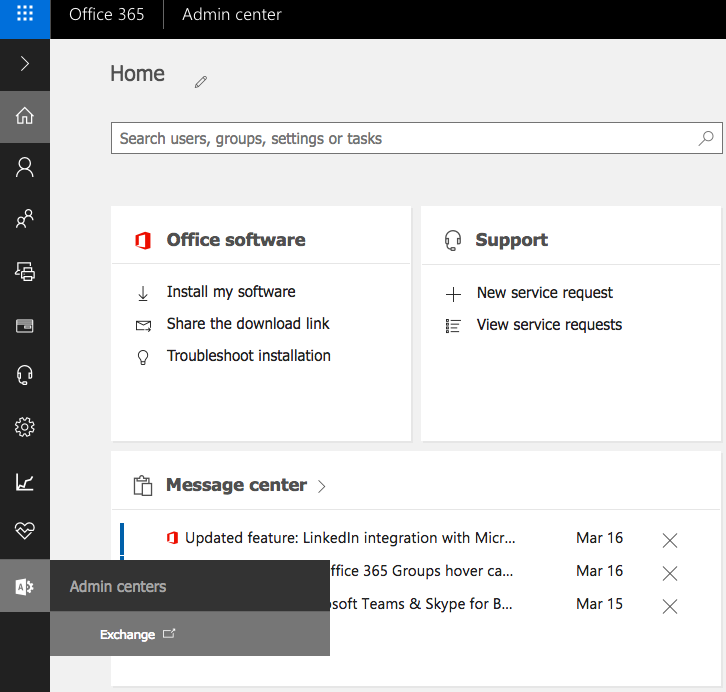This is a detailed screenshot of the Office 365 Admin Center interface. At the top left, there's a distinct blue box that acts as a header bar, clearly labeled "Office 365 Admin Center." On the left side of the screen, a vertical taskbar displays a series of icons from top to bottom: a home button, profile button, sharing button, printer devices button, a miscellaneous button, headphones button, settings button, stats button, a health button, and an admin center button.

The main section of the screen is prominently titled "Home." Near the top, there is a pencil icon and a search box that reads, "Search users, groups, settings, or tasks." Organized into three sections, the content spans the page.

1. The first section, located on the middle left, is labeled "Office software" featuring a red logo. This section offers options to "Install my software," "Share the download link," and "Troubleshoot installation."
   
2. The second section on the right is a support section, which includes two identical options: "View service requests."

3. The final section at the bottom is the "Message Center." Here, it displays an entry titled "Updated feature, LinkedIn integration with Micro..." but the text cuts off. The entry is dated March 16th and includes an 'X' icon. Below this, two more options are partially obscured by a pop-up labeled "Admin Centers." These options read "365 groups hover March 16th with an X" and "Teams and Skype for B... March 15th with an X."

The interface is designed to provide a comprehensive dashboard for managing Office 365 administrative tasks efficiently, with clear sections dedicated to software management, support, and updates from the message center.